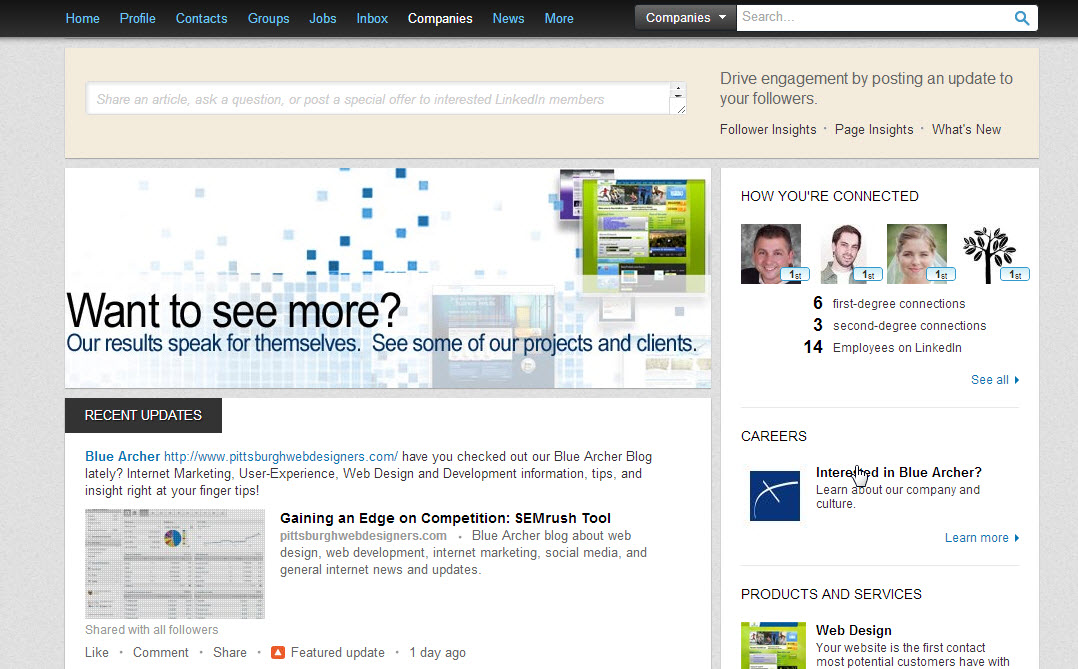The image depicts a LinkedIn website interface. At the very top, there's a black navigation bar featuring menu options in blue text: Home, Profile, Contacts, Groups, Jobs, Inbox, Companies, News, and More. Companies is highlighted in white. To the right, there's a drop-down menu and a search bar.

Below the navigation bar, there's a tan-colored area on the left with a search bar that reads, "Share an article, ask a question, or post a special offer to interested LinkedIn members." To the right of this area are options stating, "Drive engagement by posting an update to your followers," "Follower Insights," "Page Insights," and "What's New."

In the middle of the screen, on the left side, there's a white section with blue pixelated squares displaying a message: "Want to see more? Our results speak for themselves. See some of our projects and clients." Directly below this, there's a "Recent Update" section.

On the right side, there's a white box titled "How you're connected." Inside, you see a picture of a male in a black suit with dark hair, smiling. Next to him is another male with brown hair, and a beard and mustache. The third image shows a female with short brown hair, possibly wearing a veil. Below these pictures, it states: "Six first-degree connections, three second-degree connections, 14 employees on LinkedIn."

Further down, there’s a "Careers" heading with the statement, "Interested in Blue Archer," accompanied by a pointer finger icon, suggesting an interactive or clickable element preparing to engage the viewer.